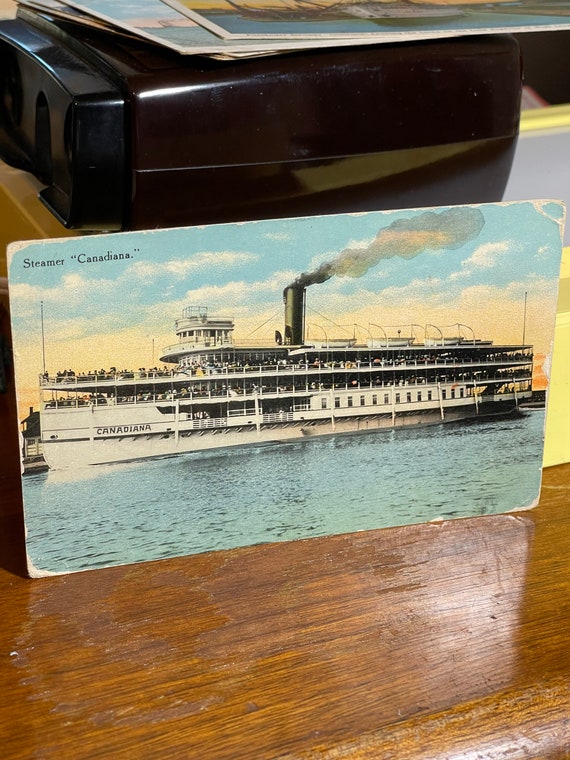The image illustrates a detailed and skillfully rendered digital artwork or drawing depicting a large, multi-deck steamboat named the Steamer Canadian. The boat, primarily white in color, boasts a prominent smokestack emitting smoke and is depicted sailing on a blue river or body of water. The sky above the boat transitions from blue to a warm orange hue near the horizon, suggesting either a sunrise or sunset, which is mirrored in the water below. This artwork is presented on a rectangular piece of material, possibly cardboard or poster board, which is resting on a dark brown wooden table against a yellow wall. Additionally, a black plastic computer printer is positioned above the artwork, with other similar pictures stacked on top of it.